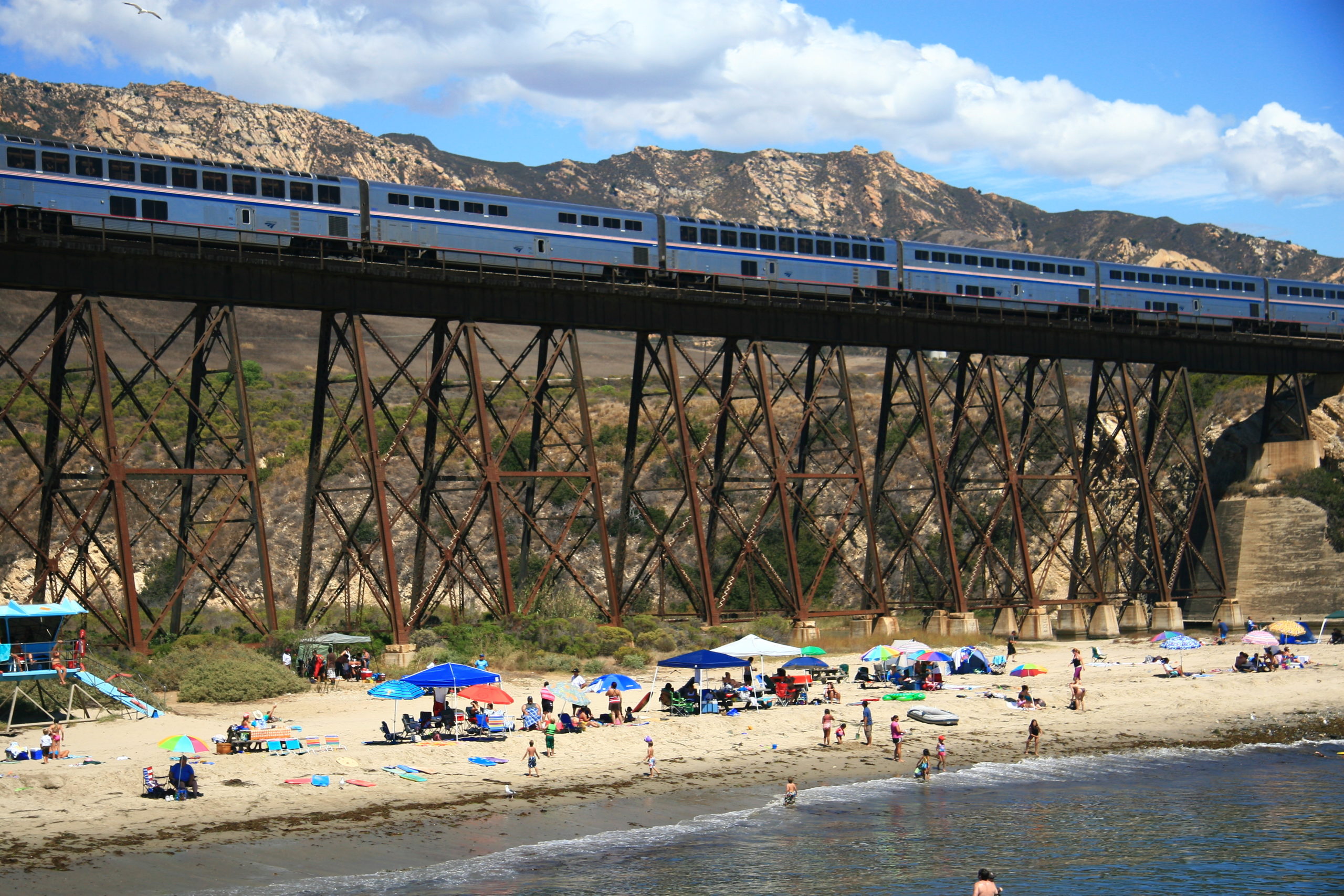This photo, taken in California during the daytime, captures a vibrant beachfront scene set against a stunning backdrop of mountains under a blue sky filled with white, fluffy clouds. The focal point is America's longest long-distance passenger train, operated by Amtrak, traveling elevated on metal beams and rocks, alongside the picturesque coastline. The beach is lively with numerous people in bathing suits, relaxing under a mix of blue, white, and green umbrellas, with coolers and air blow-up mattresses scattered across the sandy shore. In the foreground, a blue lifeguard station stands ready, overseeing swimmers and beachgoers enjoying the refreshing waters. Amidst the hustle and bustle, birds can be seen soaring in the sky, adding to the idyllic, lively atmosphere of this seaside location.